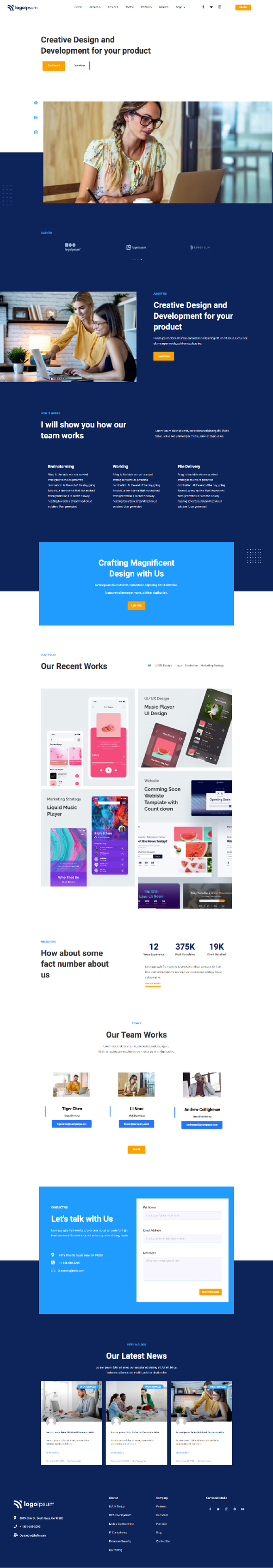The image showcases a segmented view of a website split into various sections, each designed with distinct background colors, predominantly white and shades of blue. The text throughout the image is somewhat blurry, making it difficult to read smaller details. At the top, the section features a white background with text stating "Creative Design and Development for Your Product." This section includes an image of a young woman with blonde hair styled in a braid, sitting in front of a laptop. 

Below this is a navy blue section that repeats the phrase "Creative Design and Development for Your Product" and adds, "I will show you how our team works." The subsequent section includes a light blue banner at the top with the message "Crafting Magnificent Design with Us," accompanied by an orange "Learn More" button.

Proceeding to a white background section, it highlights "Our Recent Works" alongside images of various web design pages. It also mentions "How about some fact numbers about us," displaying figures such as "12," "375K," and "19K," although the accompanying descriptive text is unclear.

Further down, the section prompts interaction with the text "Let's Talk with Us," featuring a fillable form. The bottom segment of the image, set against a darker blue background, is labeled "Our Latest News" and lists three headlines underneath.